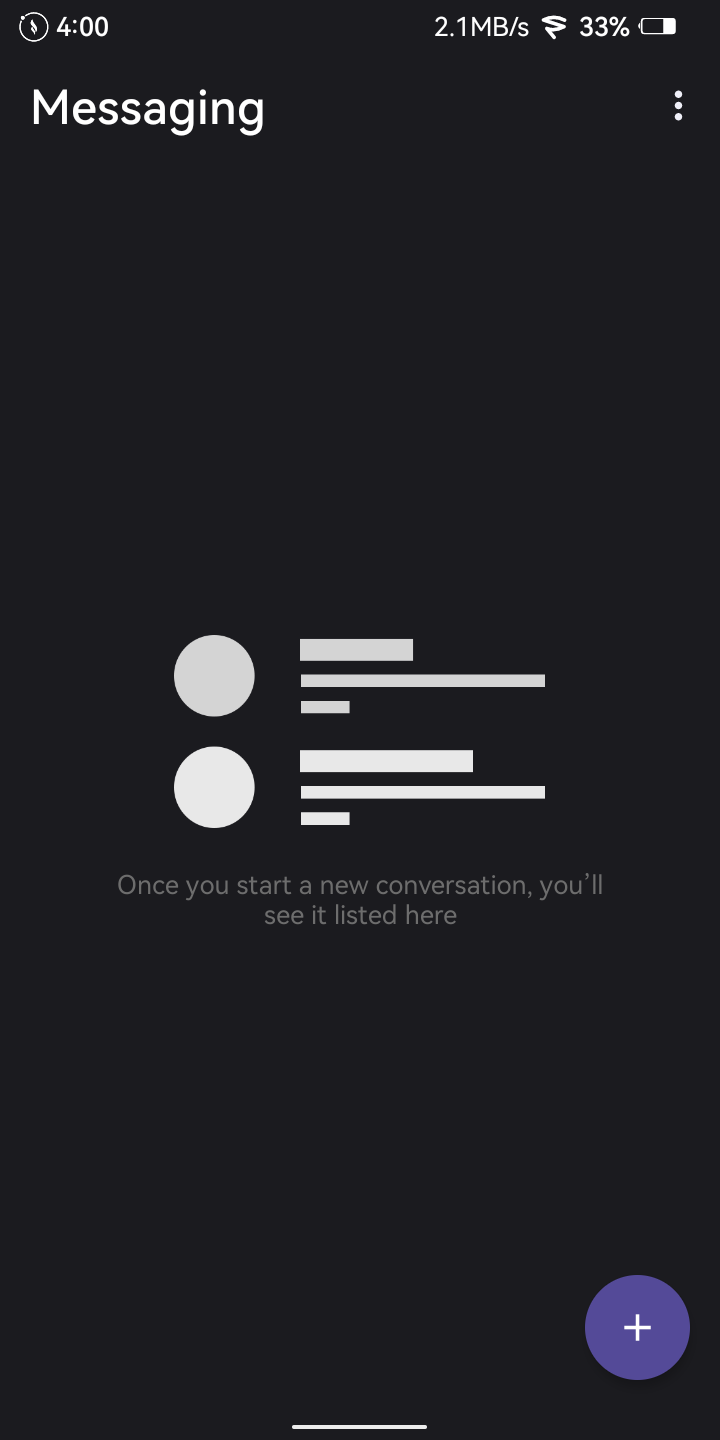The screenshot depicts a black phone screen interface, where several sections have been redacted in a grayish-white or antique white color. 

**Top Section:**
- **Time**: Displays "4:00" (possibly indicating four o'clock).
- **Data Transfer Rate**: Shows "2.1 MB/s".
- **Battery Status**: A battery icon with "33%" charge remaining.
- **Additional Icon**: A symbol resembling a lightning bolt, possibly indicating fast charging or high-speed internet connectivity.

**App Title**: In the upper left-hand corner, the word "Messaging" appears prominently in white capital letters, with a large, legible 'M'. 

**Menu Access**: On the upper right-hand side, three vertically-aligned dots indicate a button for accessing additional settings or menu options.

**Central Area**:
- **Graphic Elements**: Displays two round circles at the center, alongside horizontal lines of varying lengths: two shorter lines flanking a much longer one.
- **Notifications**: A message reads, "Once you start a new conversation, you'll see it listed here."

**Lower Section**:
- **New Message Button**: Features a round purple button with a white cross in the middle, located in the lower right-hand corner. The button color is a darker shade of purple but not too dark.
- **Indicator Line**: At the very bottom center of the screen, a line suggests the screen can be pulled down to reveal or hide a background screen similar to the design found in Apple devices.

The thoughtfully arranged elements and indications enable an intuitive navigation experience for the user.